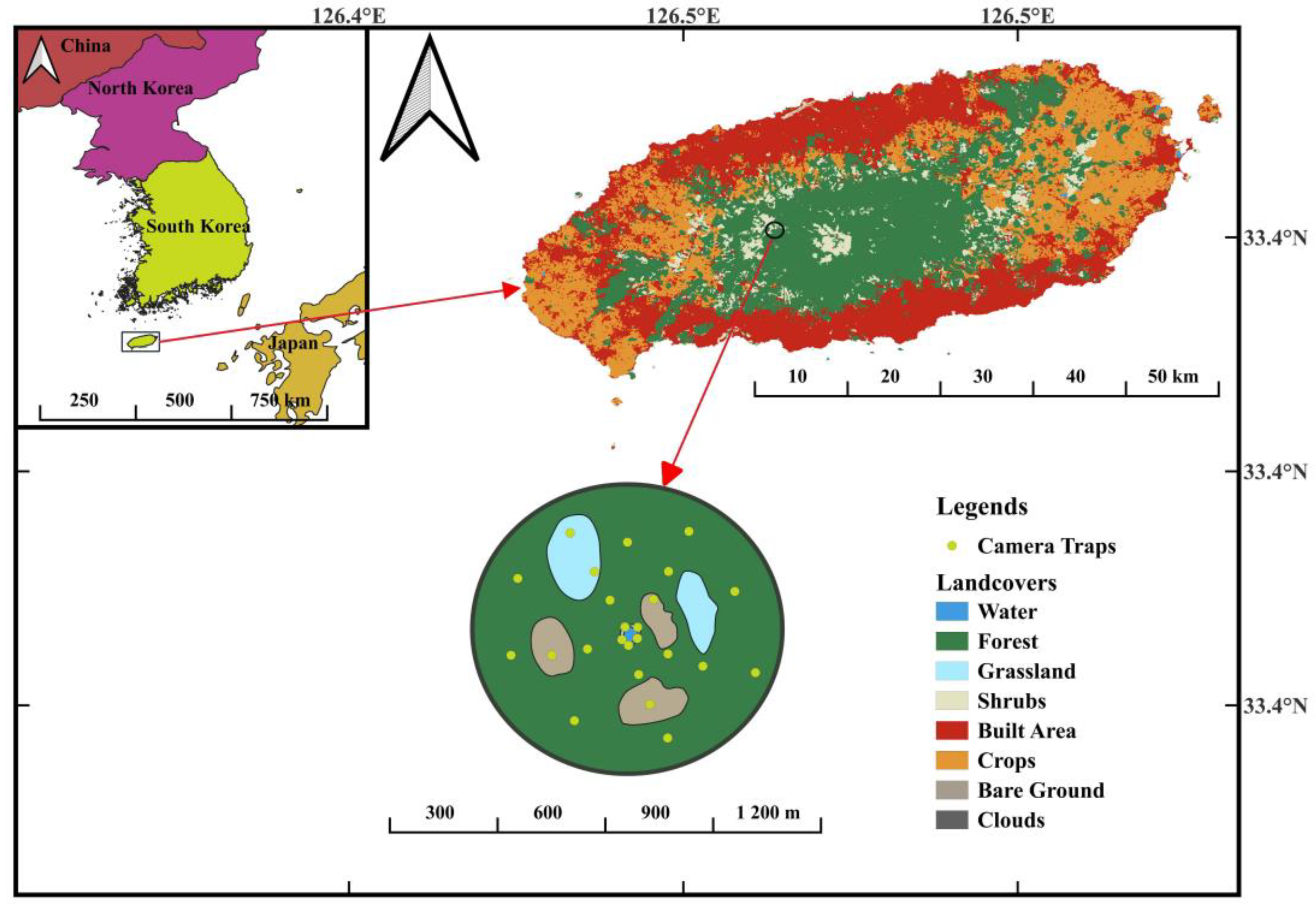The image is a detailed, multi-layered map focused on Jeju Island, located off the coast of South Korea. In the upper left corner, a political map highlights areas of East Asia, including South Korea, North Korea, part of China, and part of Japan. Jeju Island is circled and highlighted with an arrow pointing to a more detailed inset of the island on the right. The island is depicted with various color-coded areas representing different landscapes: green for forests, blue for water, red for built areas (businesses and homes), orange for crops, gray for bare ground, and white for clouds.

The map includes several scales for different levels of detail: a kilometer scale (10 to 50 kilometers) and a meter scale (300 to 1200 meters) for Jeju Island. An additional inset within this detailed map shows a further magnified section of the island, highlighting areas of forest, water, and bare ground, identified by similar color codes and small yellow dots whose specific meaning is not clarified. The map legend, found in the lower right corner, provides a comprehensive guide to the color codes used. Coordinates in black text outline the main image, adding another layer of geographical reference.